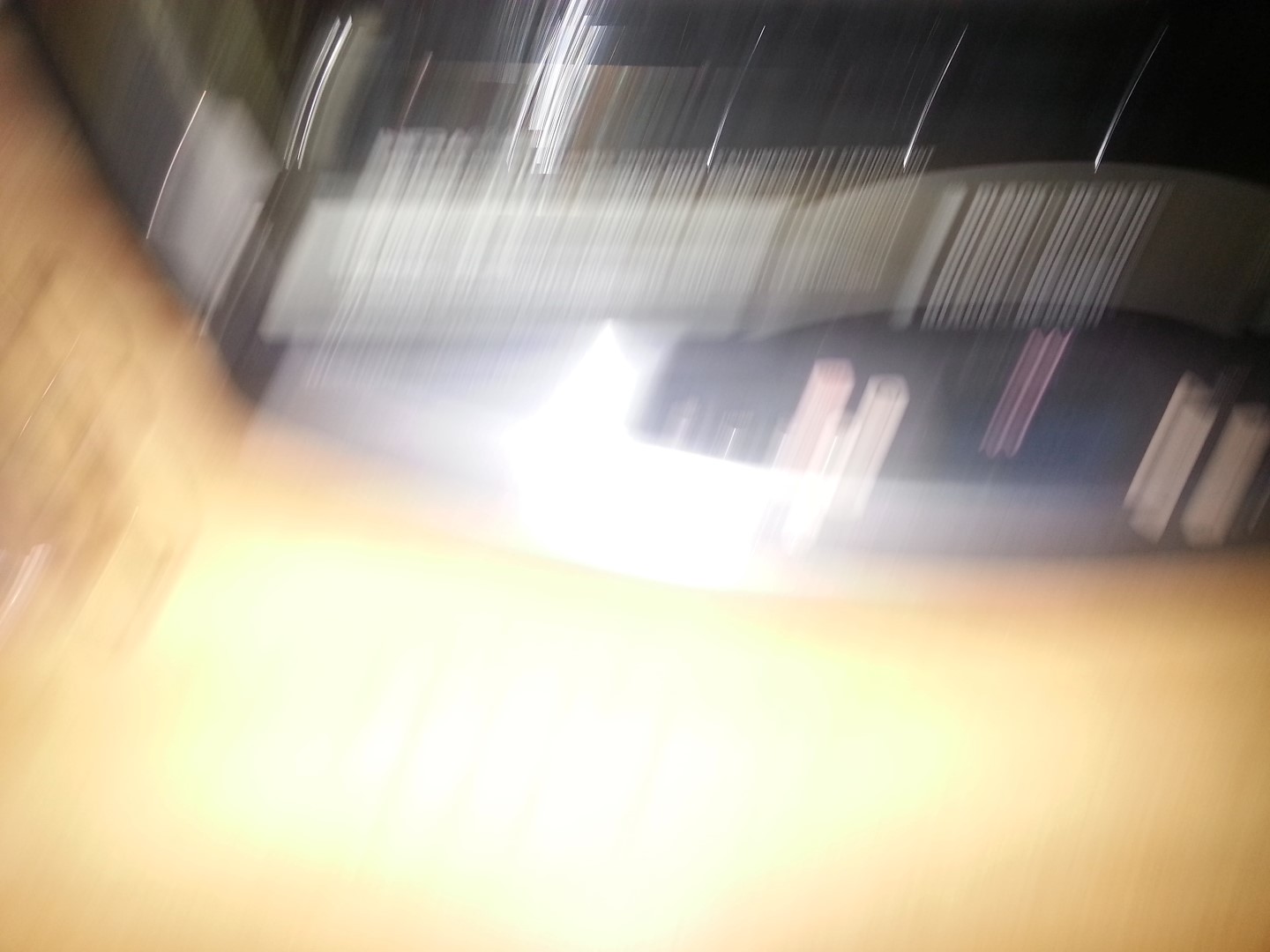The photograph is extremely blurry, making it challenging to distinguish any specific structures or figures. The bottom half of the image consists of light colors, possibly resembling flesh tones or a light source, with a pronounced glare featuring pinks, oranges, and yellows. This area forms a large, indistinct blob that tapers towards one end, suggesting possible movement. The top half of the photo is a blur with streaks of light in various colors—such as white, red, and pink—stretching vertically. These streaks could be attributed to stadium or scoreboard lights, indicating the image might have been taken at night. The background is dark blue, adding to the night-time appearance. There is a suggestion that the setting might be an elevator's interior, with potential elevator buttons to the left and brown, curved, blurry sections alongside white sections. The blurriness indicates the photograph was likely taken with a moving camera, resulting in an indistinct, chaotic image.